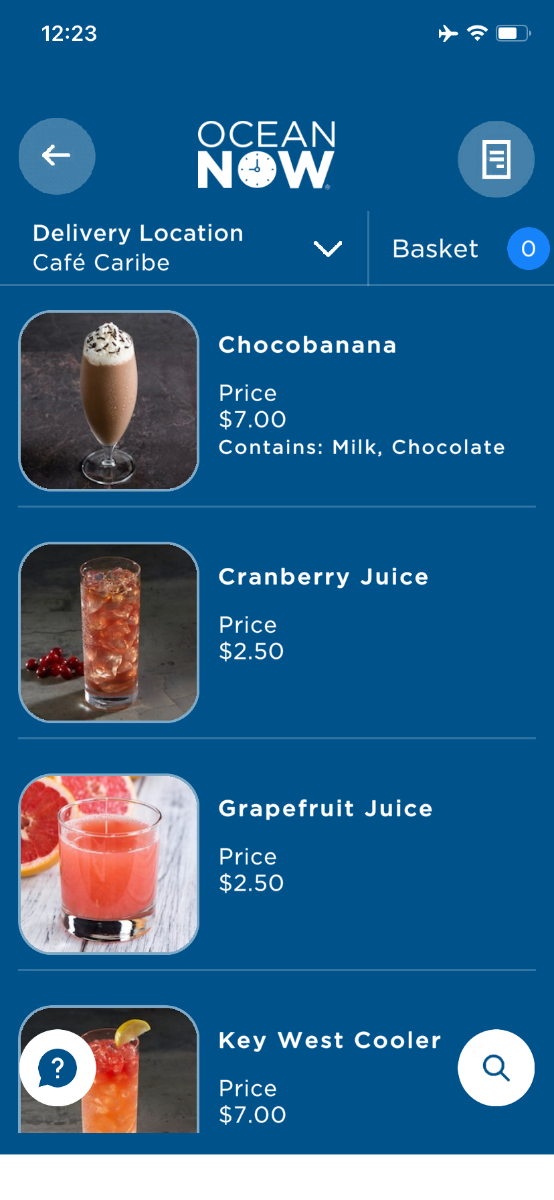**Caption: Detailed Overview of Cruise Ship Beverage Ordering App Interface**

The screenshot depicts the interface of a beverage ordering app on a mobile device, likely used on a cruise ship. In the upper-left corner, typical mobile status indicators are visible: the time reads 12:23, the device is in airplane mode, connected to Wi-Fi, and the battery is approximately 75% charged.

At the center top of the screen, the app's logo "Ocean Now" is prominently displayed. "Ocean" is in white text, while "Now" is in larger, block text with the 'O' designed as a clock showing the time of approximately 9:00. Below the logo, the current delivery location is specified as "Cafe Carib," with a drop-down menu available for changing the location. To the right, it shows an empty basket with the label "Basket 0," indicating no items have been added yet.

The screen presents four drink options, each with an accompanying image, description, price, and contents:

1. **Choco Banana**: A blended beverage served in a tall glass, topped with whipped cream and chocolate shavings. Priced at $7, it contains milk and chocolate.

2. **Cranberry Juice**: Served in a tall glass filled with ice and light cranberry juice. This drink is priced at $2.50.

3. **Grapefruit Juice**: This beverage comes in a shorter glass with no ice and is filled with grapefruit juice. It is also priced at $2.50.

4. **Key West Cooler**: Priced at $7, this drink is partially cut off by the screen. It appears to be served in a tall glass with ice and a lime garnish, featuring a mixed drink where the bottom layer is visually distinct from the top.

At the bottom of the screen, icons for a chat bot and search function are visible, suggesting options for customer service assistance or further navigation within the app.

Overall, this screenshot provides a comprehensive view of a convenient beverage ordering system designed for cruise-goers, highlighting drink choices and easy usability for guests.